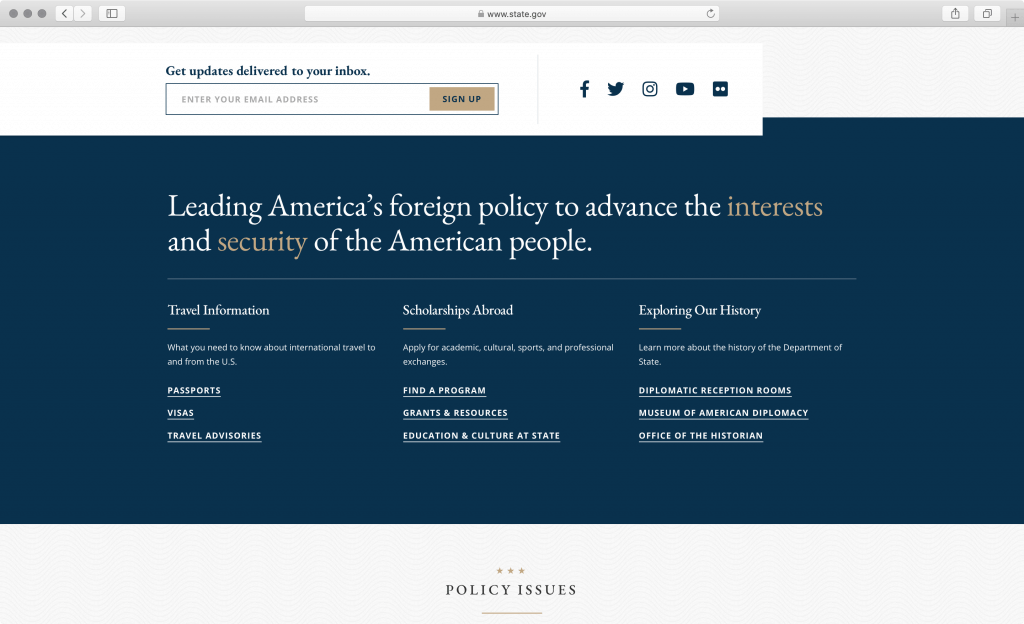This image is a screenshot of a state government website, displayed on a computer. At the very top, the URL in the browser's search bar reads "www.state.gov." Just below this, there is a subscription section with the prompt "Get updates delivered to your inbox," accompanied by a text box inviting users to enter their email address and sign up.

Beneath this section, a large, horizontal blue rectangle spans the width of the page. Inside this rectangle, white text proclaims, "Leading America's foreign policy to advance the interests and security of the American people."

Further down, the page is divided into three columns, each featuring different content:

1. **Left Column**:
   - **Travel Information** header
   - Description: "What you need to know about international travel to and from the U.S."
   - Clickable links: "Passports," "Visas," and "Travel Advisories."

2. **Middle Column**:
   - **Scholarships Abroad** header
   - Description: "Apply for academic, cultural, sports, and professional exchanges."
   - Clickable links: "Find a Program," "Grants and Resources," and "Education and Culture at State."

3. **Right Column**:
   - **Exploring Your History** header
   - Encouragement to learn more about the history of the Department of State.
   - Clickable links: "Diplomatic Reception Rooms," "Museum of American Diplomacy," and "Office of the Historian."

The website appears to be organized to provide users with clear and accessible information on various aspects of the State Department’s services and resources.